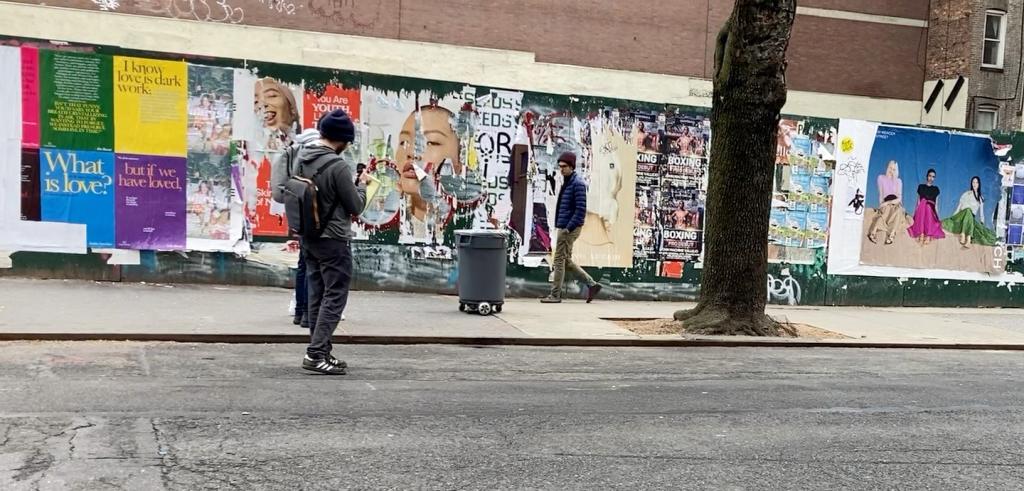The image captures a bustling urban sidewalk scene. Prominently featured is a long wall adorned with a variety of colorful posters, some depicting musicians, abstract designs, and bright phrases like "Love is Dark Work." Among these posters, one stands out, displaying images of three women in different dresses, although some of the posters appear torn and weathered.

In the foreground, a gray trash can is placed on the sidewalk. A tree with a brown trunk is seen nearby, with dirt gathered around its base. Walking past this vibrant wall, a man in tan trousers and a blue checkered shirt strides to the left, wearing a cap and glasses. Near him, another man stands wearing black pants and white and black sneakers, accessorized with a hoodie, a backpack, and a cap, seemingly engaged with his phone. A third man, also in a cap, dons gray attire but is less distinguishable. The scene offers a slice of urban life with its mix of colorful street art and everyday passerby.